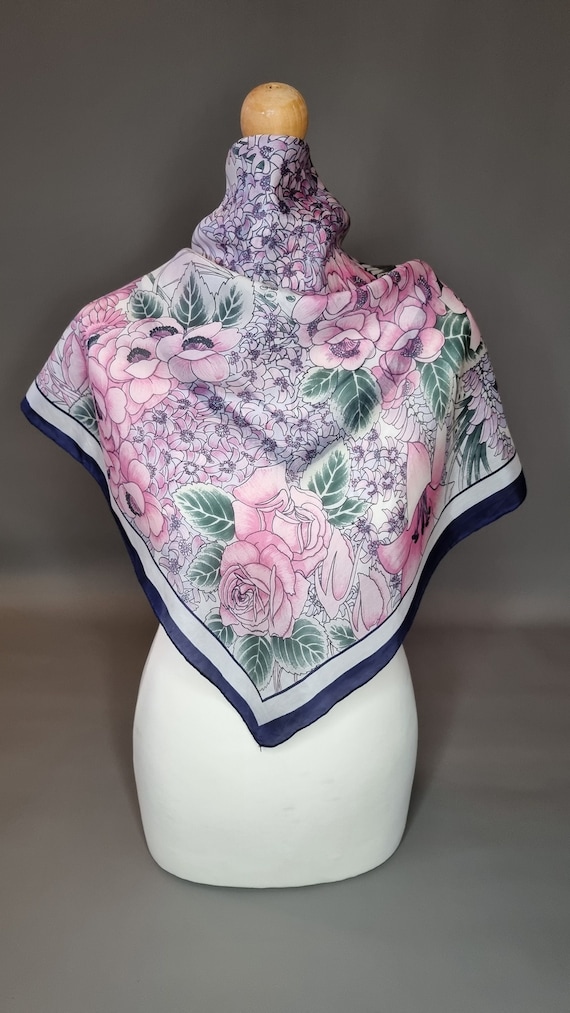This image depicts a white, torso-only mannequin, lacking both legs and arms, and topped by a wooden knob where the head would normally be. The mannequin is draped with a large, decorative scarf that entirely covers its shoulders. The scarf features a navy blue border followed by a white border, and a pattern of pink roses accompanied by green leaves. The scarf's inner portion, which appears silky, also displays clusters of pink and purple flowers, possibly including poppies. The mannequin rests on a gray surface, with a blurry, indistinct background that suggests the photo may be staged, possibly for a sales display.